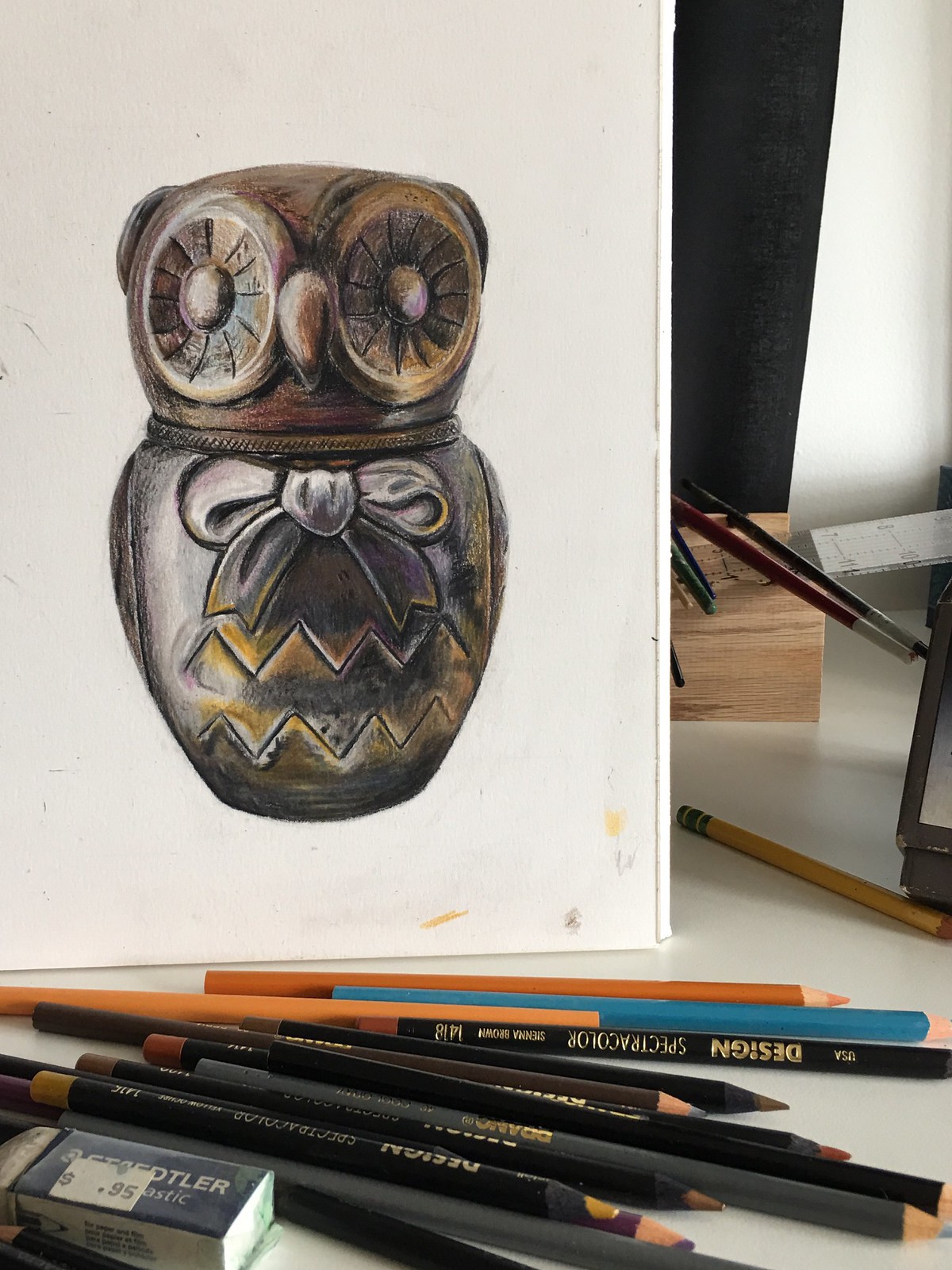The photo captures a detailed scene of an art studio workspace with various supplies arranged on a white board. Dominating the foreground are a series of Spectra Colors colored pencils arranged meticulously with their points facing right, displaying a range of shades from orange and blue to black, gray, and purple, among others. Prominently situated among these pencils is a Staedtler white eraser, marked with a 95-cent price sticker, featuring white lettering on a blue background. 

The focal point of the image is a detailed drawing of a whimsical owl sculpture, carefully rendered on white paper. This fanciful owl is characterized by its large, expressive eyes with intricate irises, a prominent beak, and rounded ears. It features a boat motif on its chest and a zigzag pattern on its lower body, reminiscent of Charlie Brown's shirt design. The coloring of the owl employs bronze, gray, yellow, and golden hues to impart dimensionality and highlight details, making it appear almost like a wooden or archaeological artifact. 

In the background, a block of wood, additional colored pencils, and part of a ruler or frame can be seen, contributing to the art studio ambiance. The image is devoid of shadows, emphasizing the vibrant details and textures of the scene.